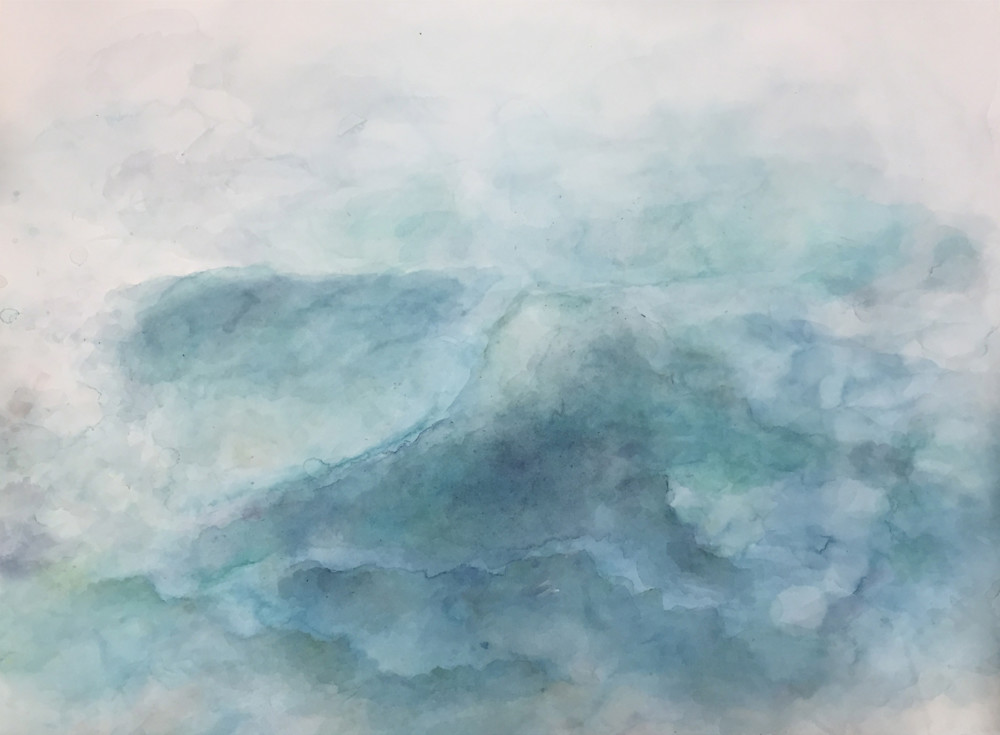This abstract image features a striking blend of colors and shapes that evoke a snowy, icy landscape. Predominantly white, the photograph is intermixed with shades of blue, green, and aqua, creating a visually captivating scene. At the top, the image is nearly pure white, with hints of off-white, gradually transitioning into a mixture of cloud-like formations and darker, more intense patches of greenish-blue towards the center. The middle of the image showcases a prominent, horseshoe-shaped mountainous range with rounded peaks, characterized by hues of blue and aqua. This mountain-like structure is surrounded by cloud-like white areas on the right and bottom right, reinforcing the illusion of a cold, frosty environment. At the bottom, the image lightens again, dominated by blue-tinted snow or ice, reflecting the icy regions reminiscent of Antarctica, Greenland, or Alaska. The entire composition, devoid of text or distinguishable objects, evokes the serene and solitary beauty of a frozen wilderness.